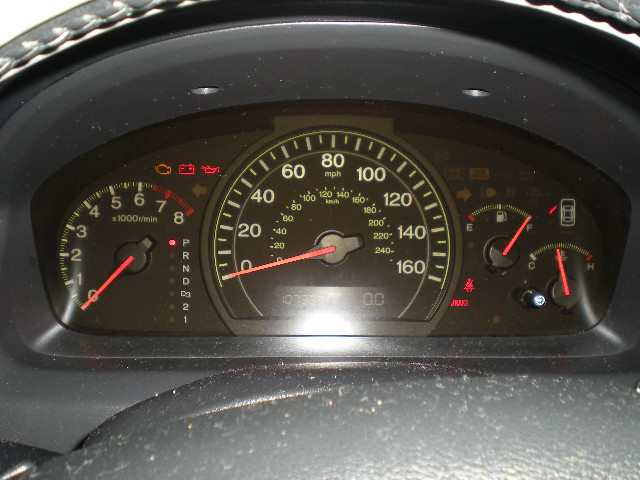This close-up image captures a detailed view of a car's dashboard, emphasizing the intricate design and various indicators. The dashboard's trim is a dark, almost black, charcoal color with a curving, arch-like top portion that rises from the lower left, peaks at the center, and dips again on the right. This arch houses two silver areas that resemble wide-set eyes overlooking the instrument cluster.

To the left, the RPM gauge features a red needle resting at zero in the lower-left quadrant. Adjacent to the RPM gauge is the transmission indicator, displaying PRND, D3, 2, and 1 in a vertical alignment, with a red light illuminating the 'P' to show the car is in park. Above the RPM gauge, three warning indicators are visible: the check engine light, battery light, and oil service light.

Central to the image is the speedometer, also at rest at zero, beneath which the car's odometer displays a reading of 107,300-plus miles. The trip meter currently reads zero. Additionally, the brake and seatbelt warning lights are both lit. The fuel gauge indicates a full tank, and there is an illuminated icon showing that the driver's side door is open. Lastly, the engine temperature gauge needle points toward the cooler side, just shy of the center, suggesting a slightly below-average engine temperature.